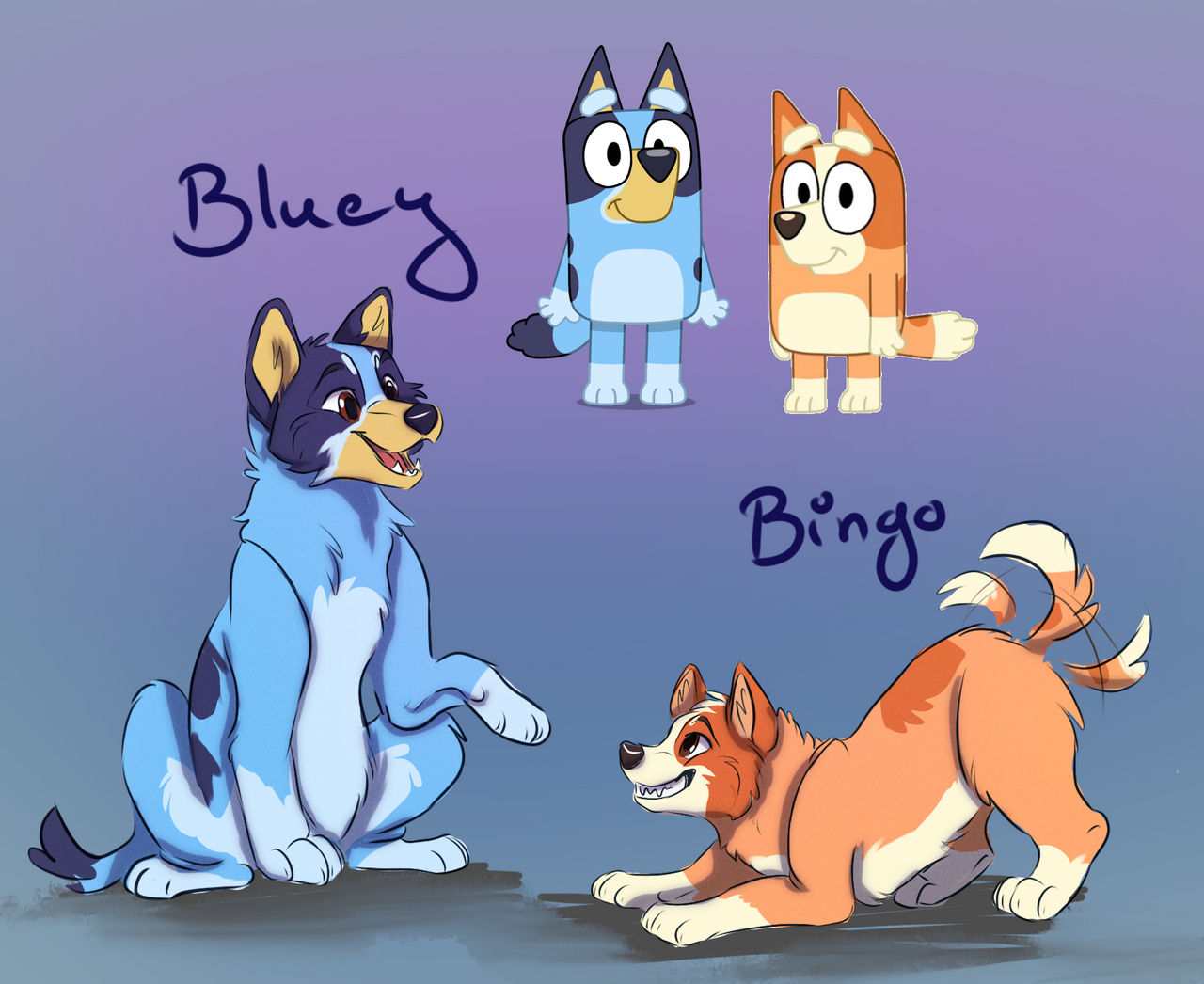This detailed fan art for the cartoon show Bluey features a gradient background transitioning from light purple to darker blue. In the top right corner, the regular cartoon versions of Bluey and Bingo are depicted standing upright, with Bluey characterized by his blue fur and Bingo by his light brown and orange fur. Below this, the image showcases more realistic, non-anthropomorphic depictions of Bluey and Bingo in a furry art style. Bluey is sitting on his haunches with an outstretched arm, while Bingo is positioned in a Downward Dog pose, with three versions of his tail indicating it’s wagging. Above the characters, their names are displayed in blue text, with "Bluey" above Bluey's head and "Bingo" above Bingo's head. The entire composition suggests a playful, fan-made homage to the beloved characters of the show.